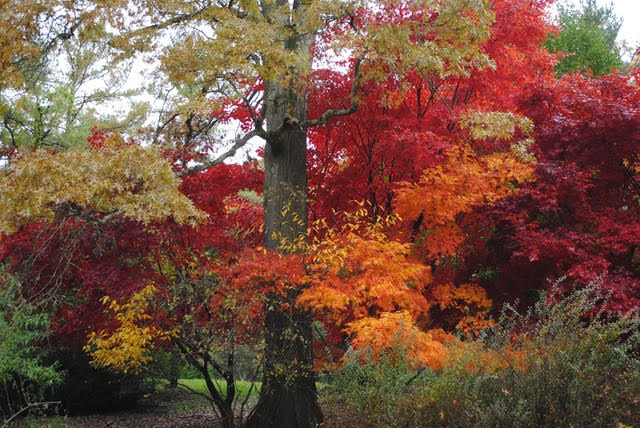This captivating image showcases a quintessential autumn scene reminiscent of a New England forest, marked by a diverse array of trees and foliage in various stages of seasonal transformation. Dominating the foreground is a tall, venerable tree with a thick trunk and an array of yellowish, cream-colored leaves. Surrounding this central tree, the foliage transitions through a kaleidoscope of autumn colors: vibrant reds, deep burgundies, golden yellows, and some lingering greens. 

On the left, a collection of thinner trees displays a mix of red and yellow leaves, while to the right and above, green leaves mingle with patches of orange, hinting at the ongoing seasonal shift. Further back, additional trees show similar transformations, with some still retaining their green hues, indicative of the slight delay in their autumnal change. 

The background features a serene meadow with green grass, providing a tranquil contrast to the vivid foliage. The sky, a stark white, suggests a crisp, cold day, enhancing the overall autumnal atmosphere. The blend of colors and textures in this close-up view of the forest captures the essence of a northeast United States landscape in full autumnal glory.